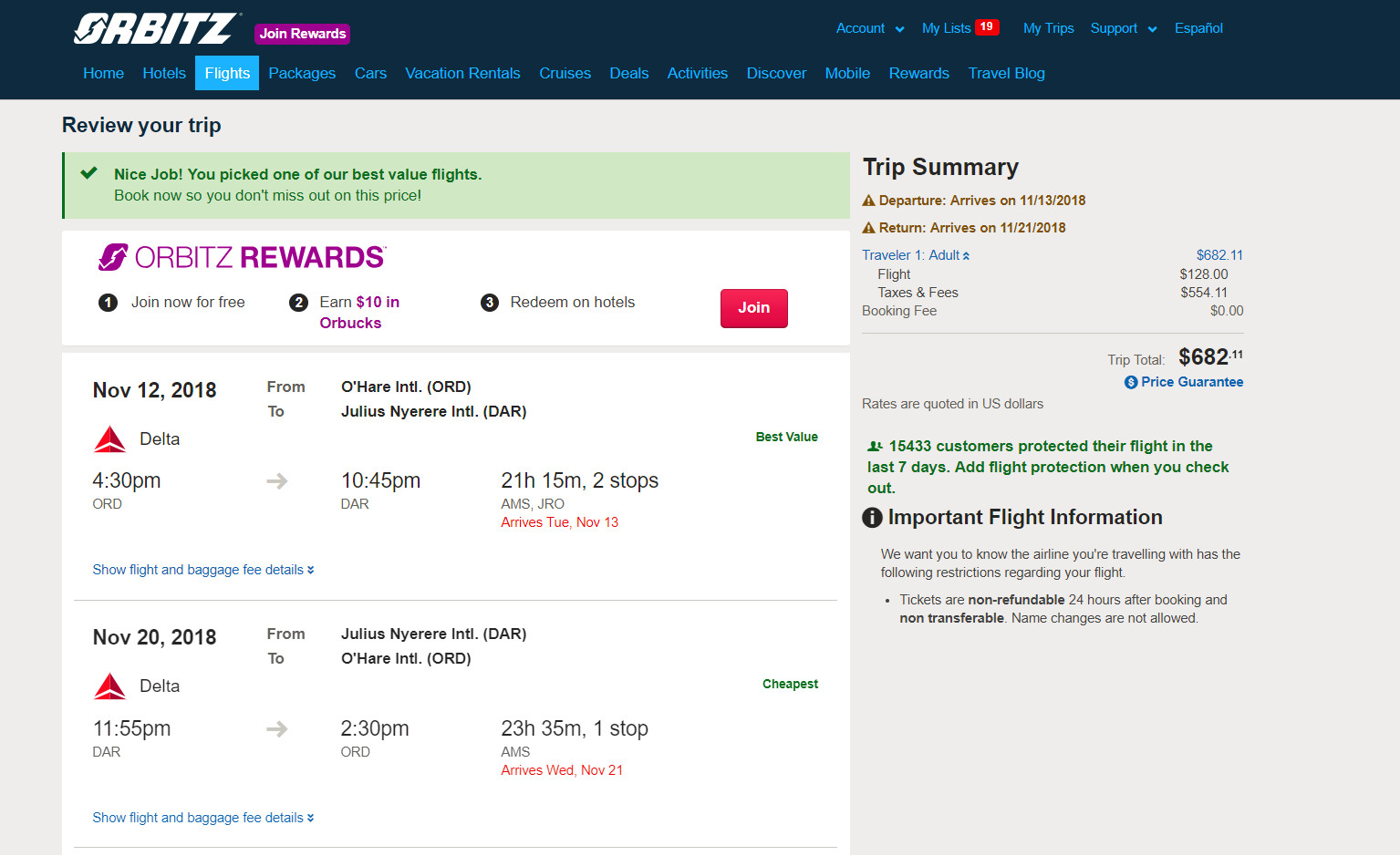The image captures a screenshot of a user's flight booking process on the Orbitz website. The user is in the "Review Your Trip" stage, examining flight details before finalizing the booking. A prominent green box at the top of the screen congratulates the user with the message, "Nice job, you picked one of our best value flights. Book now so you don't miss out on this price."

Below this, the site promotes the Orbitz Rewards program through a highlighted box that outlines the steps to join for free, earn $10 in Orbucks, and redeem these rewards on hotel stays. A "Join" button is prominently displayed to encourage immediate registration.

The selected flights are detailed further down. The outbound flight is from O'Hare International Airport (ORD) to Julius Nyerere International Airport (DAR) operated by Delta Airlines. The flight departs at 4:30 PM and arrives at 10:45 PM the next day, making for a 21-hour and 15-minute journey with two layovers: one in Amsterdam (AMS) and another in Kilimanjaro (JRO). The red text emphasizes the arrival date as Tuesday, November 13th, indicating the trip extends into the next calendar day. 

The return flight is scheduled for November 20, 2018, departing from DAR at 10:55 PM and arriving back at ORD at 2:30 PM the following day. This leg of the journey lasts 23 hours and 35 minutes with a single stop in Amsterdam (AMS). An alert in red text similarly highlights the arrival date as November 21st.

On the far right side of the screen, occupying approximately 30% of the display, the trip summary outlines the cost breakdown. The total price for the trip is $682.11. This total combines the base flight cost of $128 and additional taxes and fees amounting to $554.11. The summary also makes it clear that there are no booking fees, affirming the total price of $682.11.

This comprehensive and user-friendly interface provides a clear overview of the user's booking, flight details, and cost summary, all integral steps in confirming travel plans efficiently.